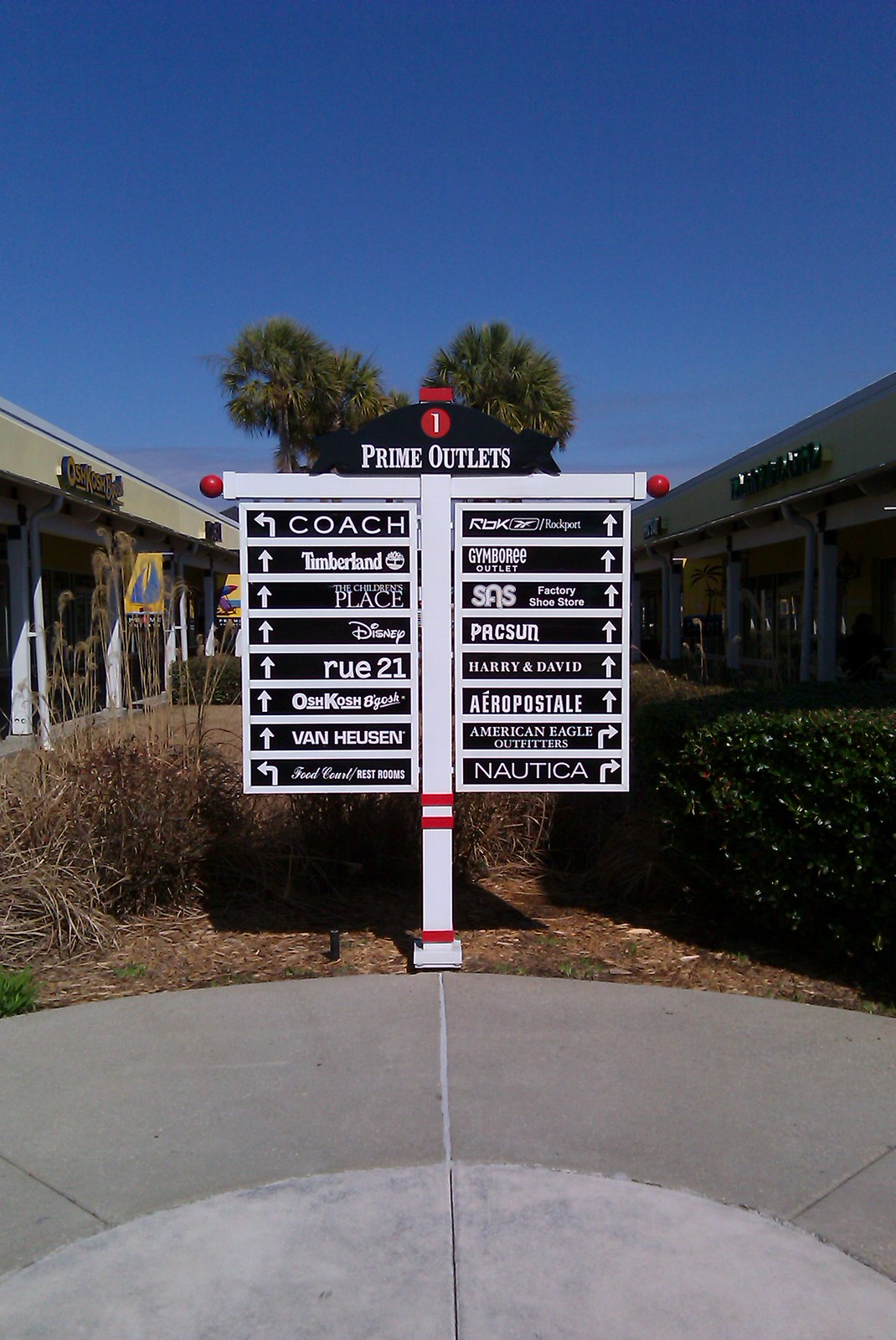In this close-up shot of an outdoor shopping development, we see a detailed sign positioned prominently in the foreground, indicating the locations of various retail stores at Prime Outlets. The sign, topped with a number one and the text "Prime Outlets", consists of a white cross structure with two black-backed billboards on either side, displaying the store names in white text along with directional arrows. Notable stores listed include Coach, Timberland, Disney, Rue 21, Van Heusen, Aeropostale, Nautica, Oshkosh, and Harry and David, though some names are partly obscured.

The bottom third of the image is dominated by a curved, concrete pathway, while a grassy, circular area with brown needles and some dry vegetation lies immediately behind. Palm trees are visible above the sign, and a clear, cloudless blue sky extends overhead, indicating a hot and dry location. Flanking the central sign, low-rise buildings of retail outlets stretch into the distance, completing the outdoor mall setting.